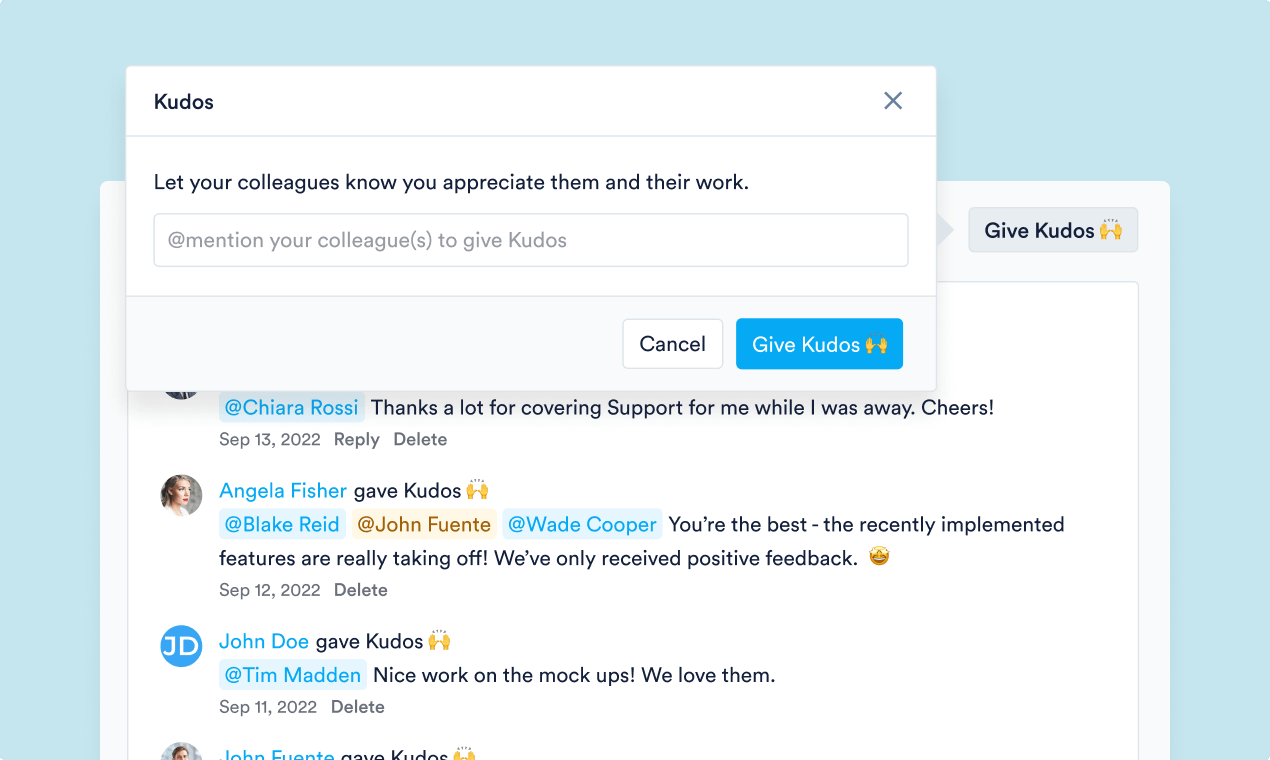A screenshot of a website displaying a series of kudos messages exchanged among colleagues. In the top-right corner, a pop-up notification appears with the message, "Kudos: Let your colleagues know you appreciate them and their work," accompanied by a text box suggesting users to "mention your colleagues to give kudos." This pop-up also features two buttons: a white "Cancel" button with black text and a blue "Give Kudos" button with white text and raising hand emojis.

Below the pop-up are three kudos messages:
1. Chiara Rossi received kudos from an unnamed colleague for covering support duties while they were away. The message reads, "Chiara Rossi, thanks a lot for covering support for me while I was away. Cheers," and was posted on September 13th, 2022. There are options to reply or delete this message.
   
2. Angela Fisher gave kudos to Blake Reed, John Fuente, and Wade Cooper, stating, "You're the best. The recently implemented features are really taking off. We've only received positive feedback," followed by a happy emoji. This message was posted on September 12th, 2022, and there is an option to delete it.

3. John Doe acknowledged Tim Madden for his excellent mock-ups with the message, "Nice work on the mock-ups. We love them," posted on September 11th, 2022. There is also an option to delete this message.

The background of the kudos messages and pop-up features a primarily white backdrop, contrasted by a light blue hue that frames the entire scene, giving a fresh and engaging look to the interface.